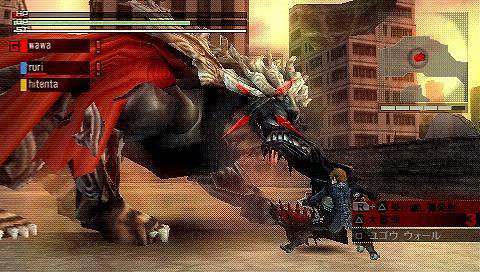This screenshot is taken from the Japanese video game "God Eater," available on the Sony PS4. The scene depicts a dramatic, apocalyptic setting with towering skyscrapers in the background and a sky that appears to be on fire, painted in hues of orange and red with smoky textures. Overlaying the image are multiple interface elements typical of a video game. 

At the top right-hand side, there is a health bar and a hit point counter, which is nearly depleted, possibly indicating the player's current health. Another health bar, likely representing the enemy’s health, is also visible. A third green bar, about three-quarters full, is situated beneath these. There is also a white bar, but its function is unclear.

Beneath these bars, Japanese text accompanies three shorter rectangular bars in red, blue, and yellow. The text likely denotes player statuses or special abilities, but due to language barriers, their exact meanings are uncertain.

In the scene, a monstrous creature dominates the right side of the image. The monster is significantly larger than the human character it faces, approximately three times the size, giving a sense of an intense battle. The creature is draped in a red cape and has prominent white horns protruding from its head. Its front limbs are large and imposing. 

The human character engaged in the fight is much smaller, dressed in a black cape or jacket and black pants, with brown hair. The disparity in size between the combatants highlights the epic nature of the confrontation depicted in the game.